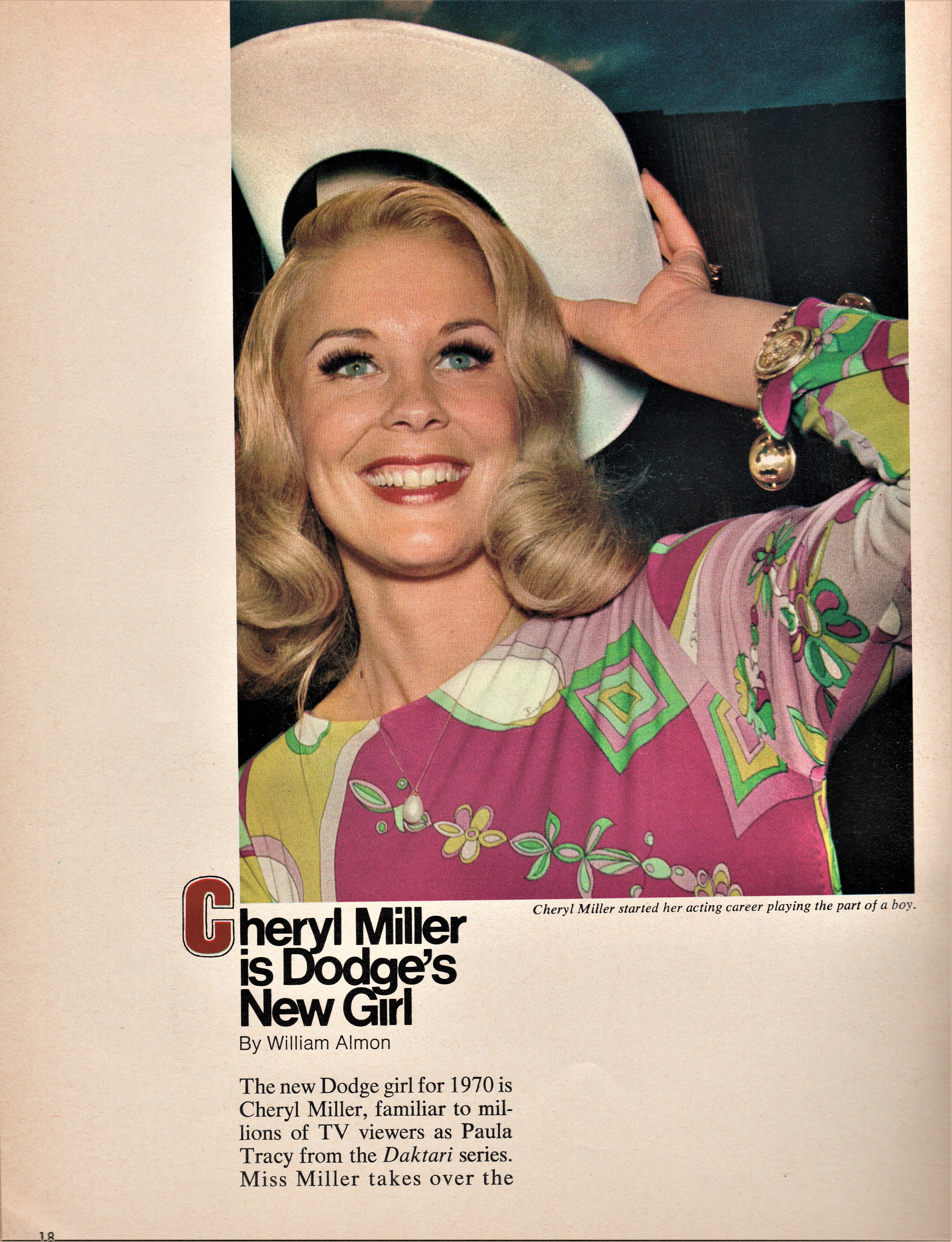The image is a photograph of a magazine page featuring a woman with shoulder-length, curly blonde hair and blue eyes. She is holding a white cowboy hat over her head and smiling brightly, with red lipstick accentuating her big smile. She is wearing a colorful floral dress in shades of pink, green, yellow, and purple, featuring both floral and square designs. Beneath the photograph, bold text declares, "Cheryl Miller is Dodge's new girl," with the 'C' in Cheryl being in red and the rest in thick black letters. Below that, in smaller text by William Almon, it reads, "The new Dodge girl for 1970 is Cheryl Miller, familiar to millions of TV viewers as Paula Tracy from the Daktari series." The background of the magazine page is an off-white color, bordered by a white outer frame. In the lower left corner, there's an indistinct page number. Additional small text underneath the main caption notes that Cheryl Miller began her acting career playing the part of a boy, although it is difficult to read.